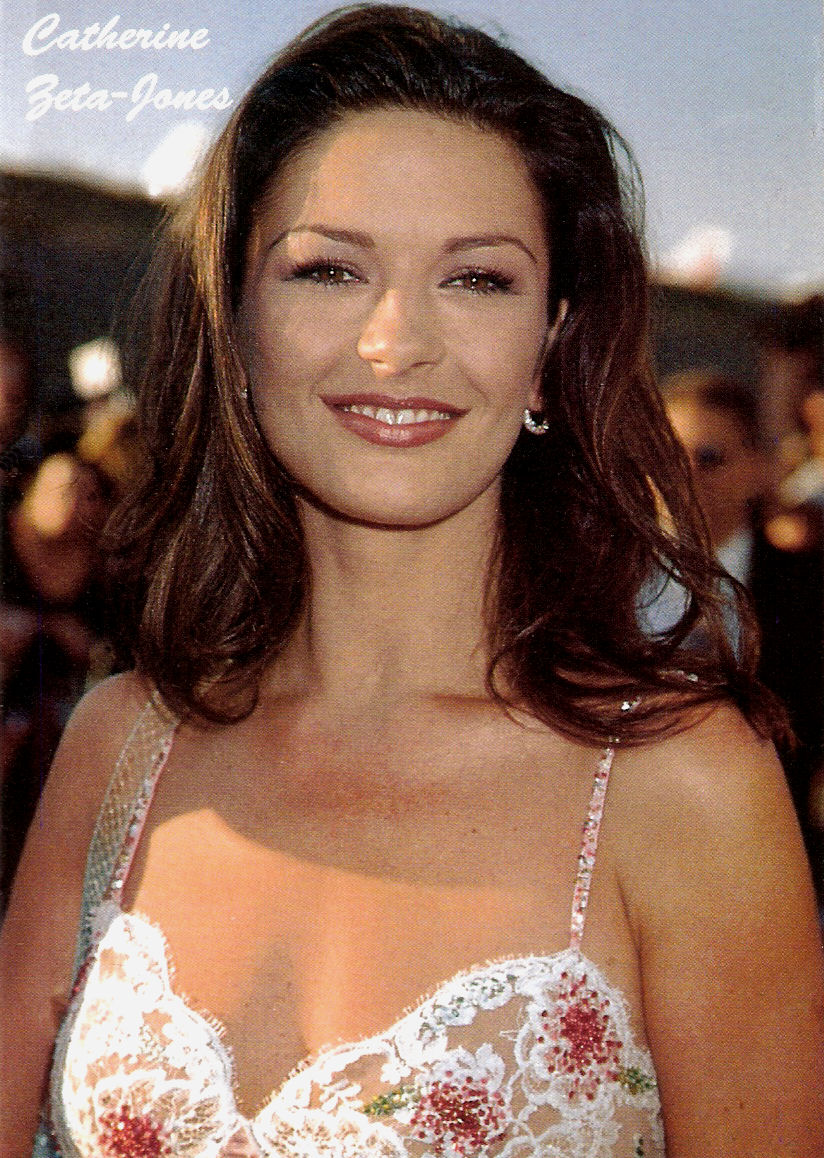This image captures a young Catherine Zeta-Jones, likely from about 20 years ago, smiling softly and looking slightly off-camera. In the upper left-hand corner of the photograph, her name appears in white letters: Catherine Zeta-Jones. She is adorned in a stunning, low-cut white lace camisole dress, detailed with red floral embellishments, hints of green, and delicate rhinestone spaghetti straps. Her outfit is complemented by a rhinestone-strap purse resting on her right shoulder and small jeweled hoop earrings. Catherine’s dark brown, shoulder-length hair frames her face, which features neatly trimmed eyebrows, brown eyes, and red lipstick that reveals a glimpse of her top teeth as she smiles. The background is bustling with suited individuals, likely photographers, adding a candid and lively atmosphere to the scene.